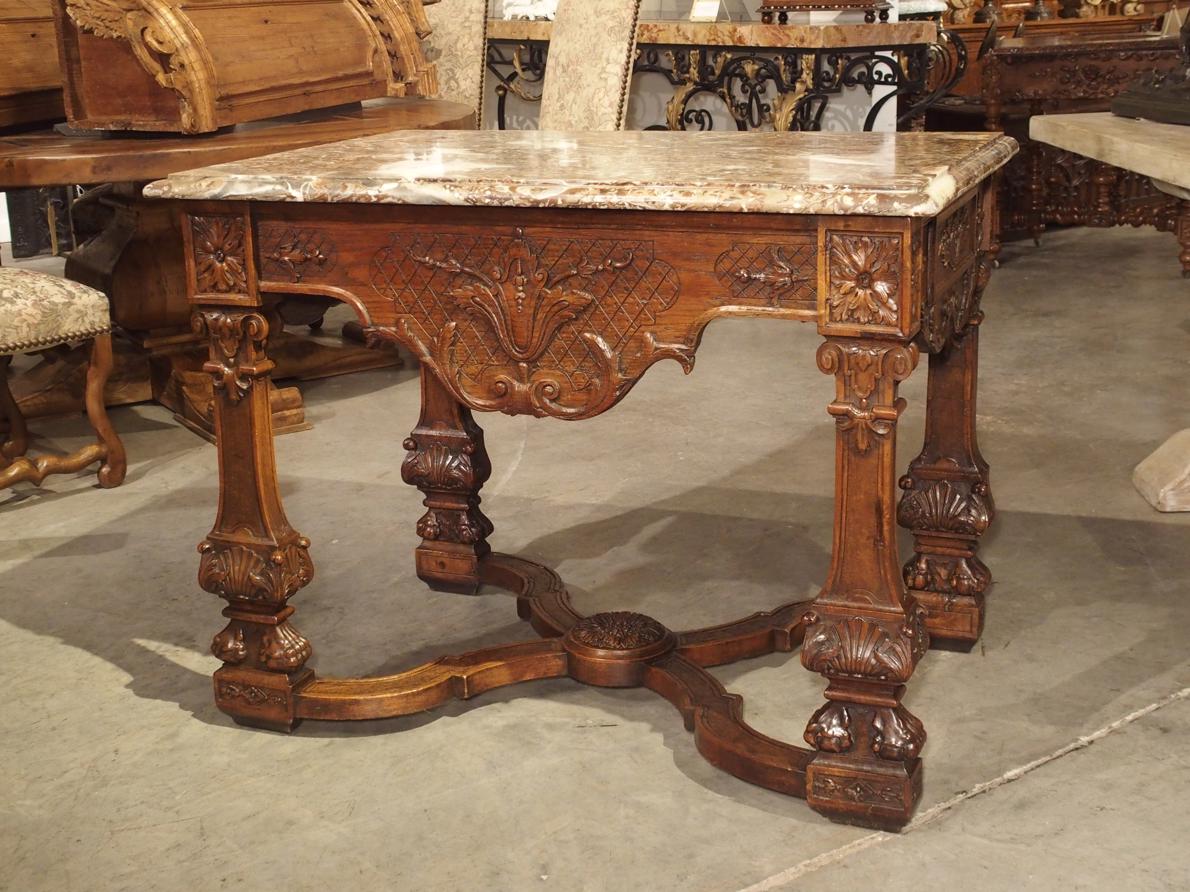This detailed photograph showcases an indoor setting filled with various pieces of antique furniture. Central to the image is a mid-height, intricately designed wooden foyer table. The table features a glossy brown finish and a prominent, polished marble top. The marble surface, an elegant blend of brown and ivory with curved edges, stands out with its unique patterns of white and darker brownish-yellow veins. The table is supported by four legs, each masterfully carved, and connected by a crisscross structure at the base, adding to its antique charm. 

The floor beneath the table is made of concrete and is colored in a tannish gray hue, casting dual shadows towards the left and back of the table due to the overhead lighting. Flanking the central table, the background reveals more antique wooden furniture, including what appears to be a roll-top desk perched atop a heavy, round wooden dining table. Also visible are partial views of chair seats and legs, suggesting their upright stance behind the central table, and another marble and iron table further back. Adding to the visual complexity, there is an indeterminate wooden piece and a marble tabletop with a pedestal foot peeking from the right side of the picture. The entire room exudes a rich historical ambiance, enhanced by the interplay of light and shadow.